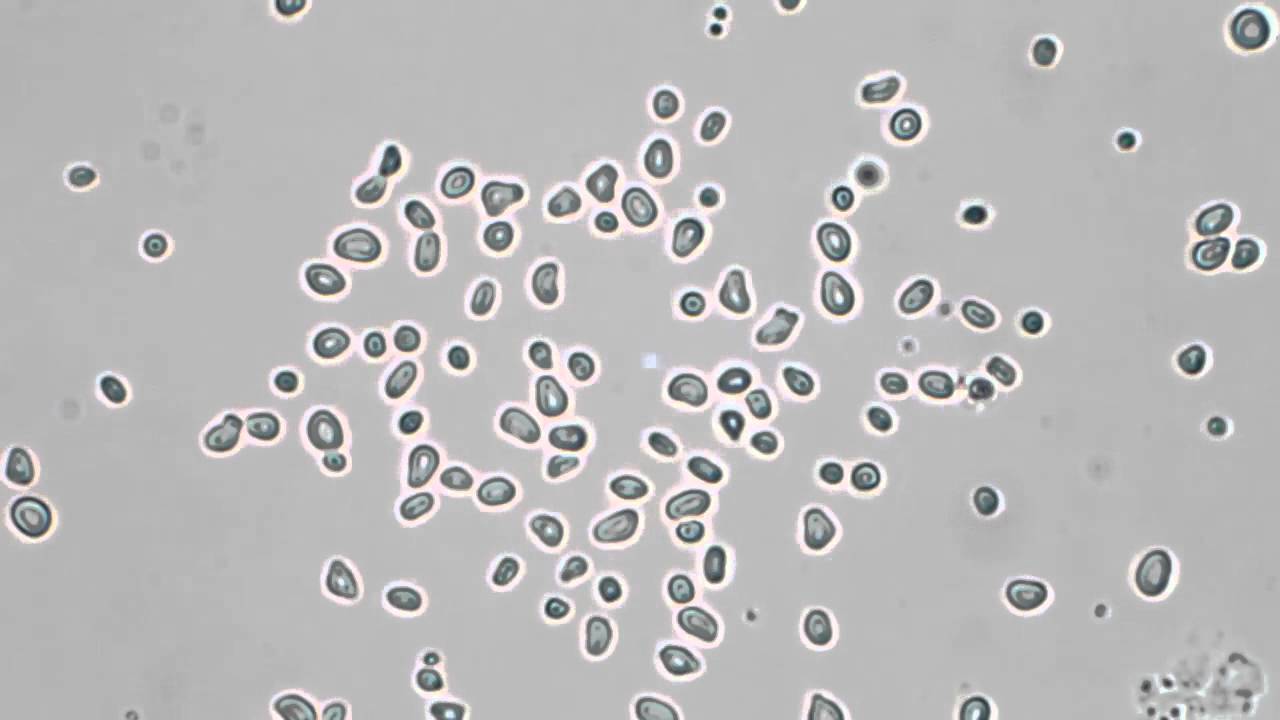This image displays a microscopic scene in a horizontal rectangle format, featuring numerous round and oval structures on a very light gray to off-white background, reminiscent of a slide under a microscope. The grayscale picture includes various sizes of these objects, with some clustered densely in the center and gradually spacing out towards the edges. The structures, possibly cells or small parasites, exhibit both circular and oblong shapes. Many of these entities bear a resemblance to half-sliced avocados or red blood cells, characterized by enhanced borders and a central divot, all surrounded by a white outline. The overall palette is devoid of color, emphasizing the grayscale and highlighting the detailed, intricate forms captured in the microscopic view.